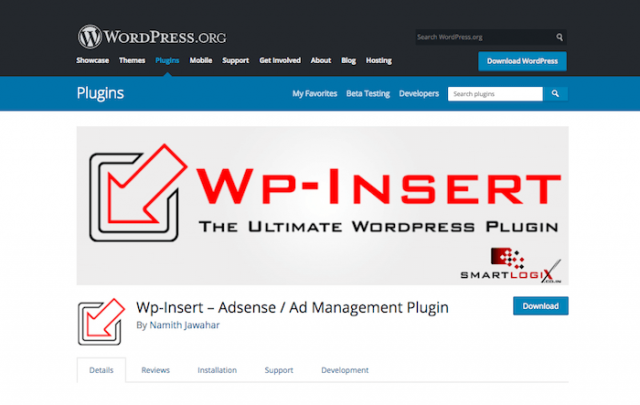Screenshot from the WordPress.org website showing the WP Insert Plugin:

The image captures a desktop view of the WordPress.org website. It prominently displays the interface with various navigational drop-down menus such as "Showcase," "Themes," "Plugins," "Mobile Support," "Get Involved," "About," "Blog," and more. 

In the top-right corner, there is a search bar accompanied by a magnifying glass icon. Below this, a blue button labeled "Download WordPress" is visible. Further down, there are additional tabs and options including "Plugins," "My Favorites," "Beta Testing," and "Developers," along with a specific search bar for plugins.

Dominating the center of the screenshot is a large graphic featuring a red triangle and a red arrow inside a square. The graphic highlights the "WP Insert" plugin, described as "the ultimate WordPress plugin" for AdSense and ad management, created by Namith Juhar. Accompanying this description, there is a conspicuous blue "Download" button along with supplementary tabs labeled "Details," "Reviews," "Installation," "Support," and "Development."

The website's design features a sleek black border at the top, followed by a blue section, and the rest of the page incorporates a clean white background, creating a visually appealing and user-friendly interface.